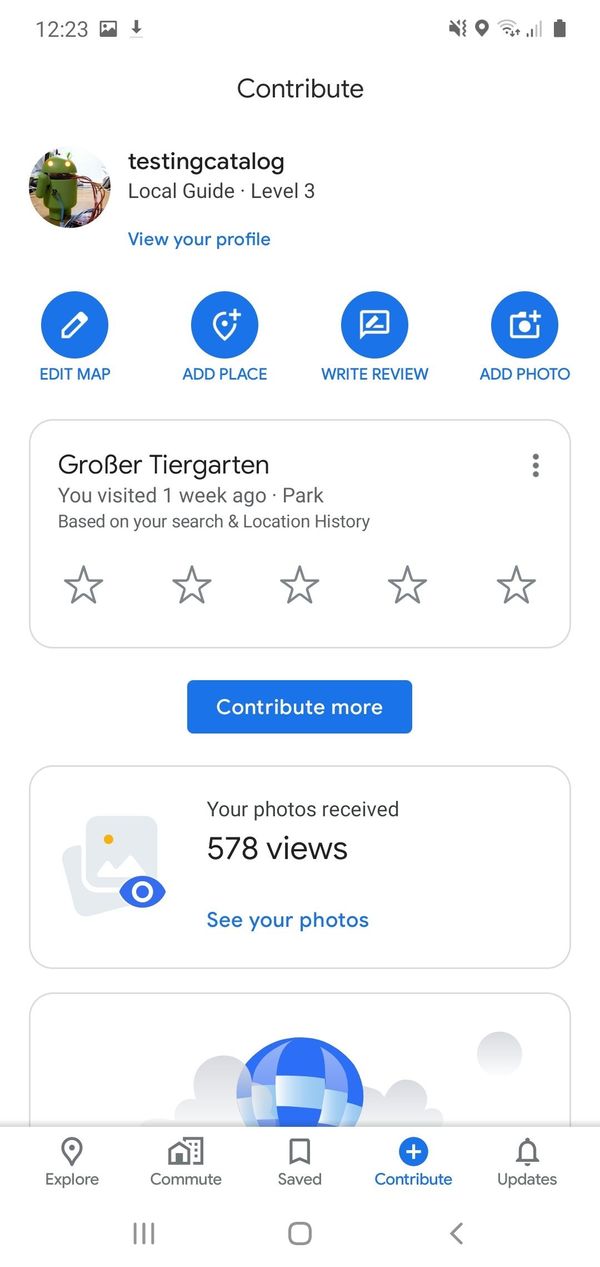**Detailed Caption:**

A screenshot of a cell phone screen taken at 12:23, as indicated by the time displayed at the top. The standard set of five icons is positioned at the top right corner of the screen. Directly below the icons, the word "Contribute" is prominently shown in black text with a capital "C". 

Beneath "Contribute," there is a circular profile picture or avatar adjacent to text that reads "Testing catalog" in black. Next to this, the phrase "Local Guide • Level 3" is displayed. Below it, the blue link text "View your profile" can be found.

Following this section, there are several interactive buttons, each designed with a corresponding icon inside a blue circle. The buttons are labeled "Edit map," "Add place," "Write review," and "Add photo."

Further down, a highlighted rectangular box contains the text "Grobertier Garten," indicating a park visited one week ago. This information appears based on the user's search and location history. Beneath this text, there are five blank stars for a rating, and to the side, a blue "Contribute more" button is available.

At the bottom of the screen, another rectangular box displays the message "Your photos received 578 views." This section includes an icon of two overlapping squares and a blue link reading "See your photos."